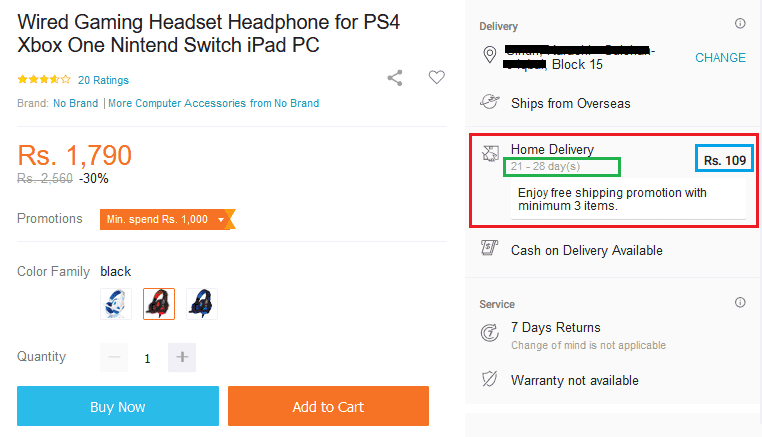This image showcases a Wired Gaming Headset Headphone designed for compatibility with various devices including PS4, Xbox One, Nintendo Switch, iPad, and PC. Situated prominently on the right side of the image, there is a vertical box labeled "Delivery". Within this box, the "Home Delivery" option is highlighted with a red square outline, indicating that home delivery will take between 21-28 days. Additionally, there is a blue outlined square around the price tag, RS.109, located in the upper right corner of the Home Delivery section. The box also features a promotional message in black font stating, "Enjoy free shipping with a minimum of 3 items."